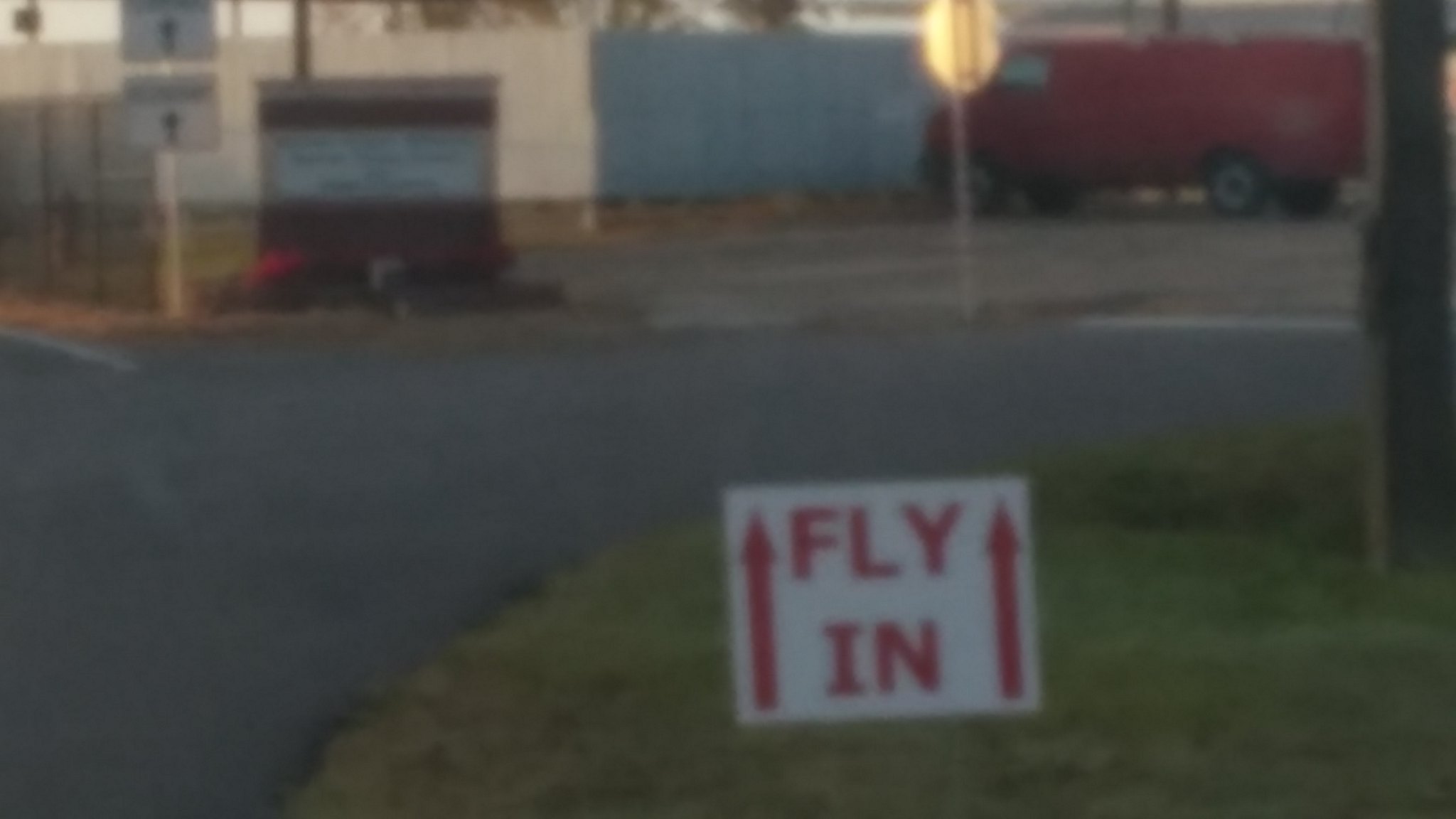In this grainy, vintage outdoor photo, a scene captures a small patch of vibrant green grass surrounded by a curved black asphalt road, resembling a four-way intersection. Prominently placed in the grass is a white sign with red letters reading "Fly In," accompanied by two black arrows pointing forward. Adjacent to this area, a red van is parked near a building with a light-colored top and dark brown bottom, featuring a garage door and a small parking lot. The surroundings include a stop sign, a brick sign adorned with pink flowers, and a fence with another white, unreadable sign. Scattered wooden crates with white boxes sit near the lush green trees visible in the background, hinting at the edges of the location.